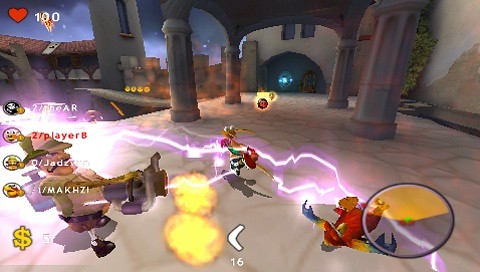The video game still captures intense kinetic action set in what appears to be an Italianate or Mexican-style villa with distinctive stucco roofs, gray cylindrical columns, and stone floor pathways. The central focus is a cartoonish character in the left foreground, distinguished by a handlebar mustache and a distinctive hat, possibly a deerstalker or a pith helmet. He wields a ray gun in his right hand, from which two lightning bolts emanate, one striking towards the center and the other branching towards the lower right of the image. The background architecture features arches and a tall gray structure with a window, characteristic of a second-story villa. 

Within the frame, there are multiple action elements: several indistinct video game-ish figures in combat, a character resembling a red chicken or parrot with multicolored wings lying prone in the foreground, and two orange puffs of fire to the left of center. Additionally, a purple lightning bolt adds to the vividly dynamic scene. The interface displays various game elements, including names like Player B, Jadz, and Makizzi, a visible gold dollar sign in the bottom left corner, and a red heart with the number 100 in the upper right corner. Icons and scores are aligned along the left image edge, enriching the immersive gaming experience.